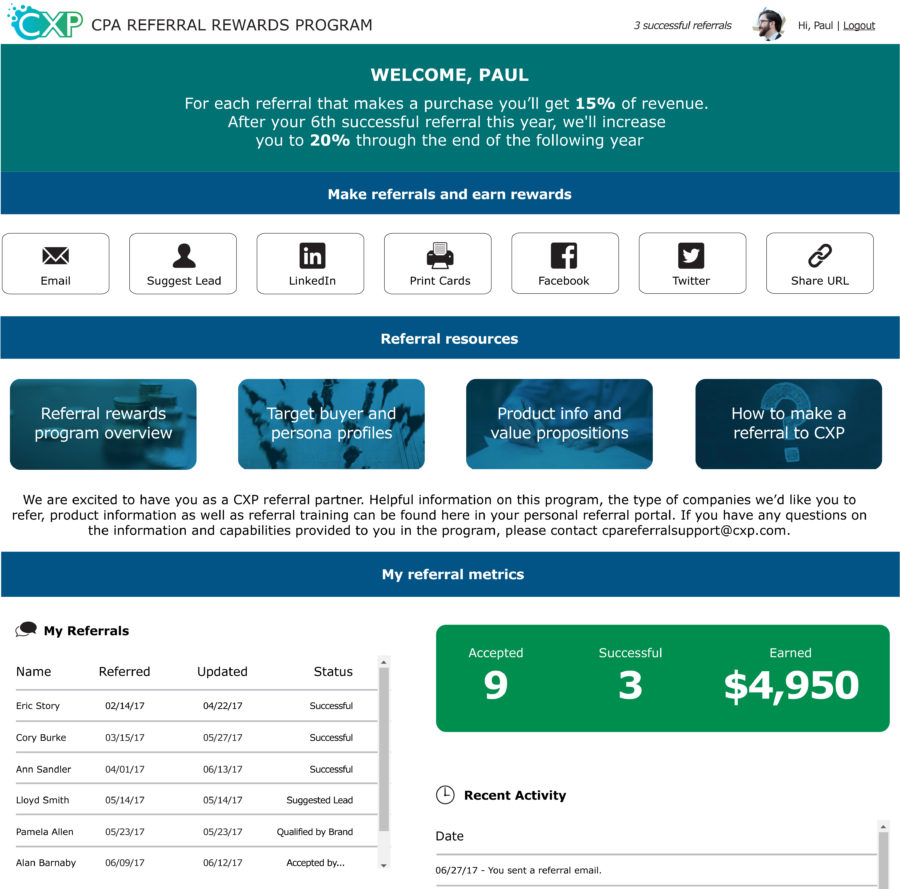The image depicts a screen capture of a website interface for the "CPA Referral Rewards Program." In the upper left corner, a logo for "CXP" is prominently displayed against a gradient background transitioning from blue to green, with white lettering.

On the upper right, there is an account login section displaying the user's profile picture, featuring a man with peachy beige skin, European facial features, black hair, and a chinstrap beard. Next to the profile, it indicates that the user has made "three successful referrals."

Just below, a welcome message reads, "Welcome, Paul. For each referral that makes a purchase, you'll get 15% of revenue. After your sixth successful referral this year, we'll increase you to 20% through the end of the following year."

Beneath this, a section titled "Make Referrals and Earn Rewards" lists several methods for making referrals, including email, suggest lead on LinkedIn, print cards, Facebook, Twitter, and share URL.

Further down, another section provides an overview of the referral rewards program. It includes sub-sections such as "Referral Rewards Program Overview," "Target Buyer and Persona Profiles," "Product Info and Value Propositions," and "How to Make a Referral to CXP." The text describes how excited they are to have the user as a referral partner and explains that helpful information on the program, the type of companies to refer, product information, and referral training can be found in the personal referral portal. For queries or information, users are directed to contact support via "CPAReferralSupport@cxp.com."

At the bottom of the screen, referral metrics are displayed. The dashboard shows various categories such as "Referred," "Updates," "Status Successful," or "Suggested Lead," and "Qualified by Brand." The metrics indicate that the user has made nine accepted referrals, out of which three were successful, earning over $4,950 from the referral program.